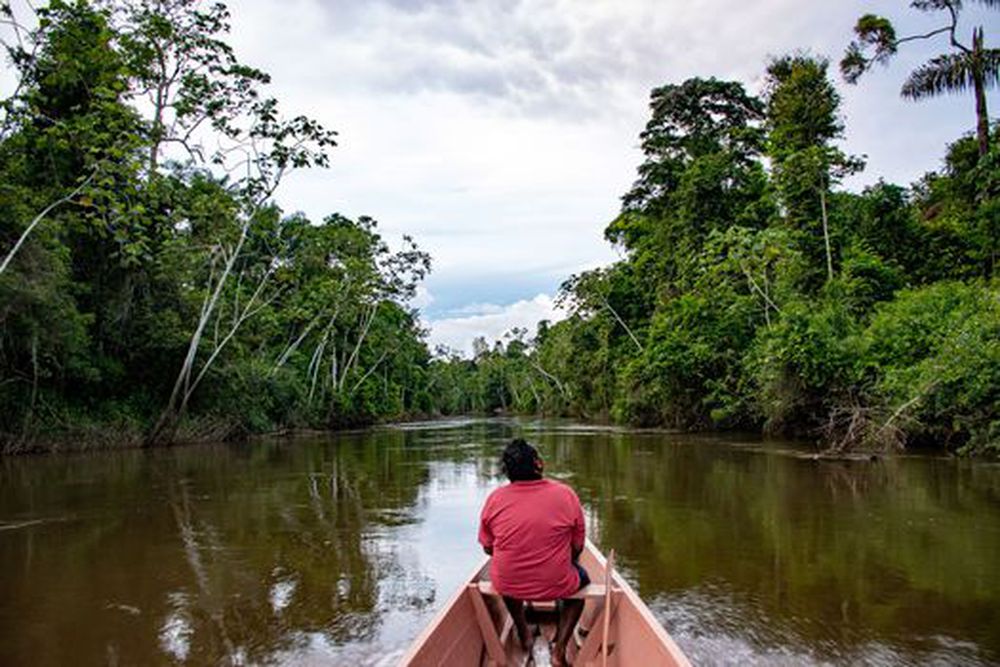In this vibrant and detailed scene, a person sits in a wooden boat, resembling a canoe, navigating down a seemingly endless river flanked by lush, green trees on both sides. Captured from behind, the individual wears a pinkish-red t-shirt and shorts. Their dark skin contrasts with the bright surroundings. They appear to be gazing upwards towards an overcast sky, which, despite heavy clouds, reveals patches of blue, indicating a bright mid-day. The river appears brownish-green and reflects the dense foliage along its banks. No other boats are in sight, and the serene waterway, although not particularly high, stretches out invitingly, offering ample space for exploration. The scene's tranquility is enhanced by the absence of paddles, suggesting peaceful drift down the river.